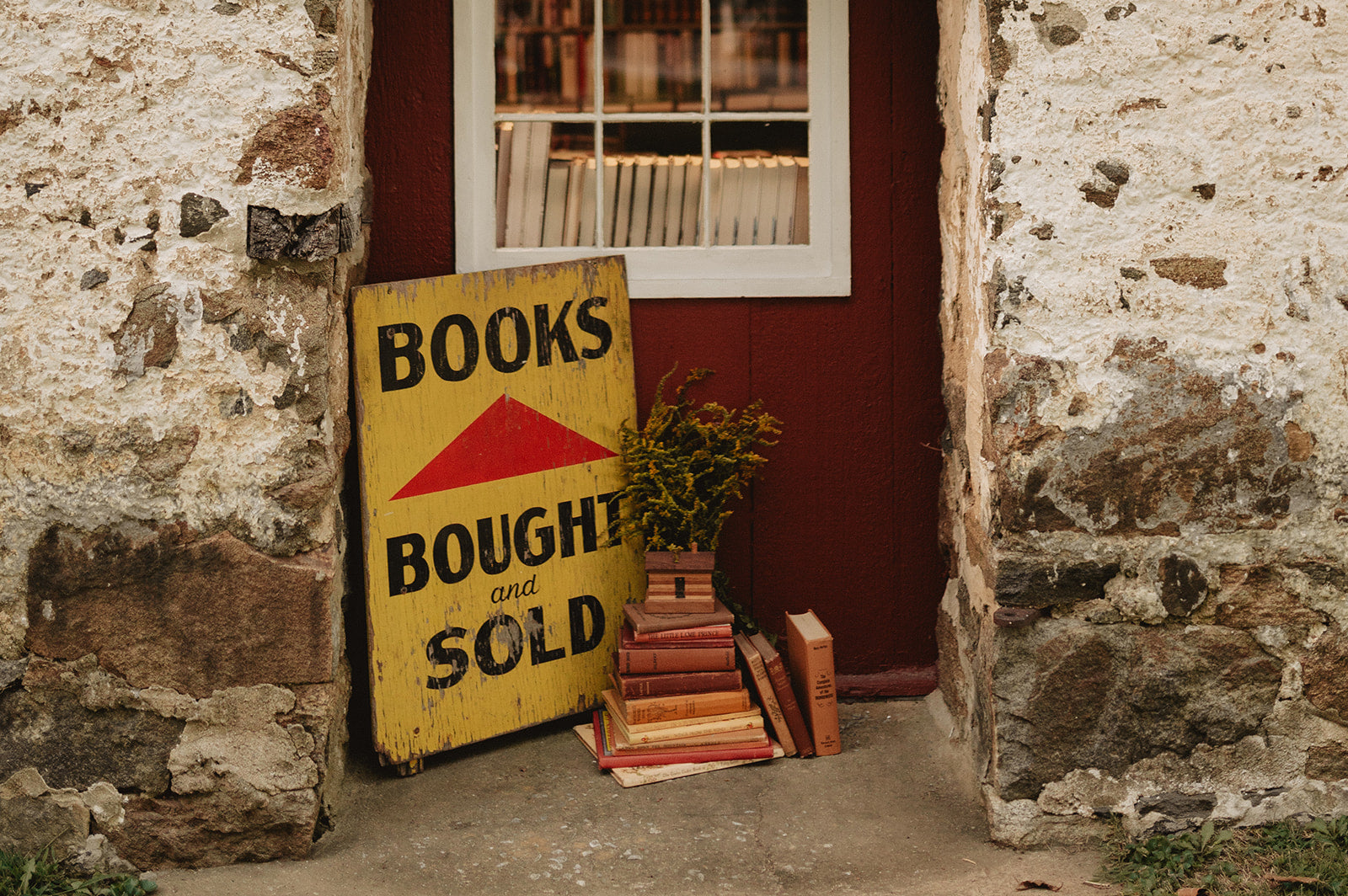This photograph captures the charming entrance of a rustic bookshop nestled in a stone building. The entryway, framed by weathered white stone walls with patches revealing the underlying gray and dark brown rocks, features a maroon wooden door with a six-pane white-trimmed window at its center. Flanking the doorway, and partially in front of the window, are stacks of books arranged both vertically and in a leaning fashion, their colors ranging from orange to red. These tomes create a triangular structure, culminating in a small potted plant at the top. To the left of the door, an antique yellow wooden sign with a red triangle arrow prominently declares, "Books Bought and Sold." The combination of cracked stucco, exposed stone, and the scatter of literary treasures evokes a timeless and inviting atmosphere, perfect for book lovers. Through the window, more books can be seen lined up inside, adding to the cozy allure of this quaint, literary haven.